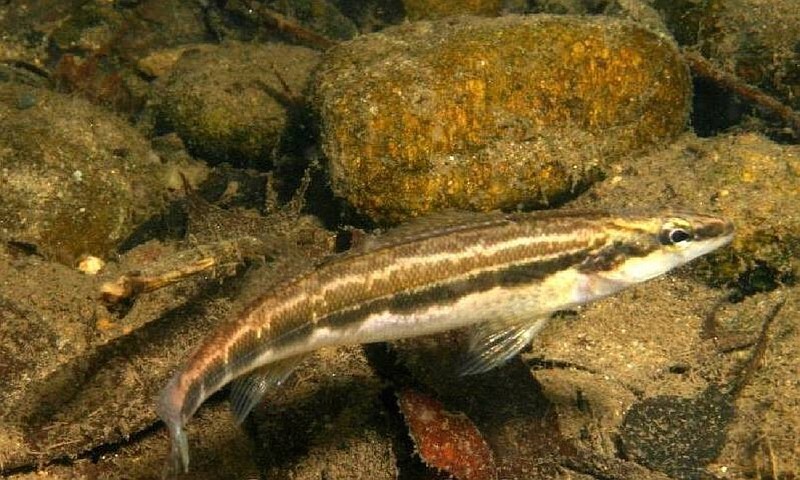This detailed image captures a rare and exquisite sickle darter fish (S-I-C-K-L-E-D-A-R-T-E-R) underwater. The fish, distinguished by its long, narrow body, dominates the frame, swimming to the right. Its underbelly glows with a luminescent white hue, contrasting sharply with the ornate, complex pattern of brown and beige scales on its back. A prominent dark stripe runs along its side, extending from the eye to the nose, giving it a unique and recognizable appearance. The semi-transparent fins and pointy face add to its delicate allure. Behind the fish, the underwater floor features a rustic array of moss-covered rocks, boulders, and twigs, with a mix of sand and other underwater elements. The overall scene has a brown and green mossy tone, emphasizing the natural habitat of the sickle darter and adding depth to the clean, clear underwater photograph. Despite the murky, plant-like growth on the rocks, the clarity of the image beautifully highlights the intricate details of the fish, making it a captivating shot of this rare aquatic marvel.